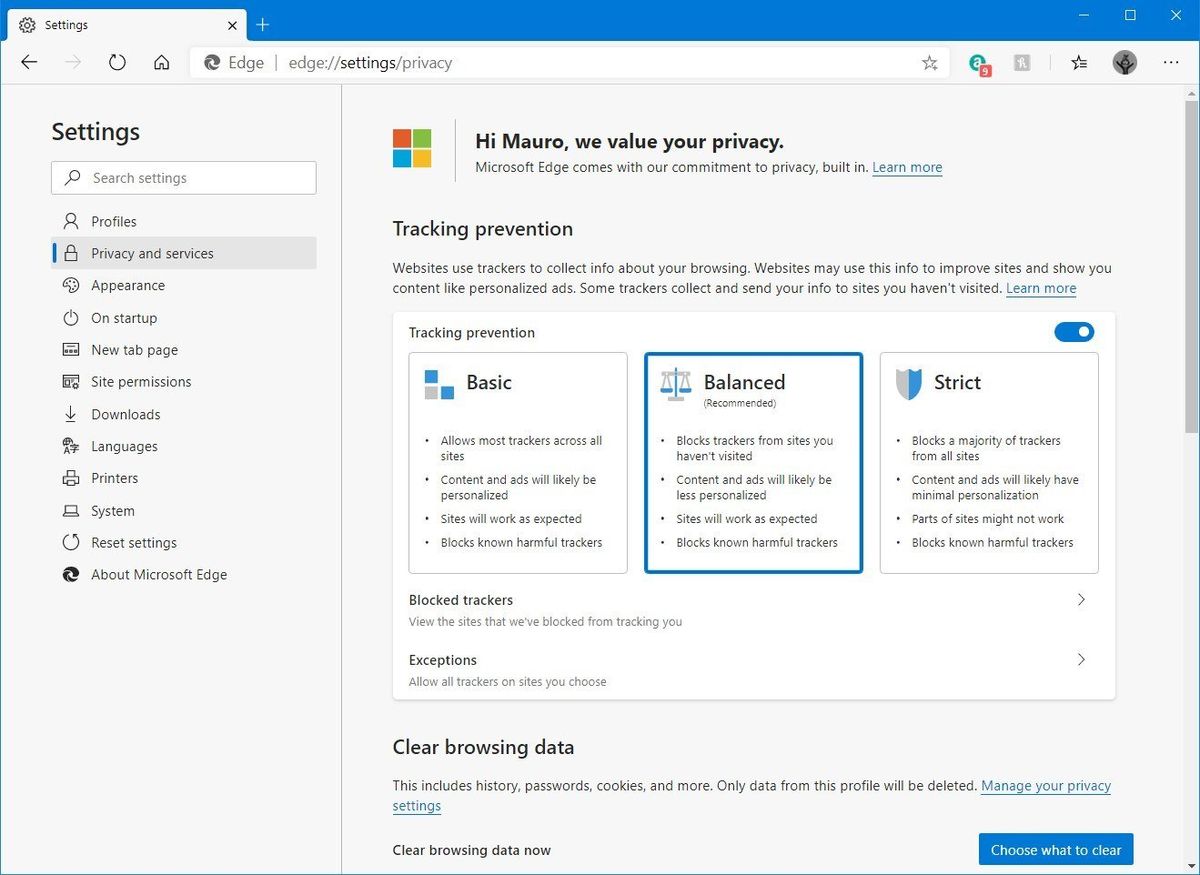Certainly! Here is a more detailed and cleaned-up caption for the image:

---

This image displays the privacy settings page of the Microsoft Edge browser. At the top, it greets the user, "Hi Maro," and assures the value of privacy. The main heading reads "Edge Settings - Privacy."

The section titled "Tracking Prevention" explains that Microsoft Edge is committed to privacy with built-in tracking prevention features. It details how websites use trackers to gather information about your browsing habits, which can be used to improve sites and deliver personalized ads. Some trackers may also gather data from sites you haven’t visited.

A clickable blue link labeled "Learn More" is available for additional information.

The middle section of the page features three levels of tracking prevention settings: Basic, Balanced, and Strict. Each option provides different degrees of tracker blocking and user data protection.

Additionally, there is a section titled "Clear Browsing Data," which outlines that users can delete history, passwords, cookies, and more. It specifies that only data from the current profile will be deleted. At the bottom, there is a link labeled "Manage your privacy settings" for further customization.

---

This cleaned-up caption provides a clear and comprehensive description of the content and layout of the privacy settings page in Microsoft Edge.